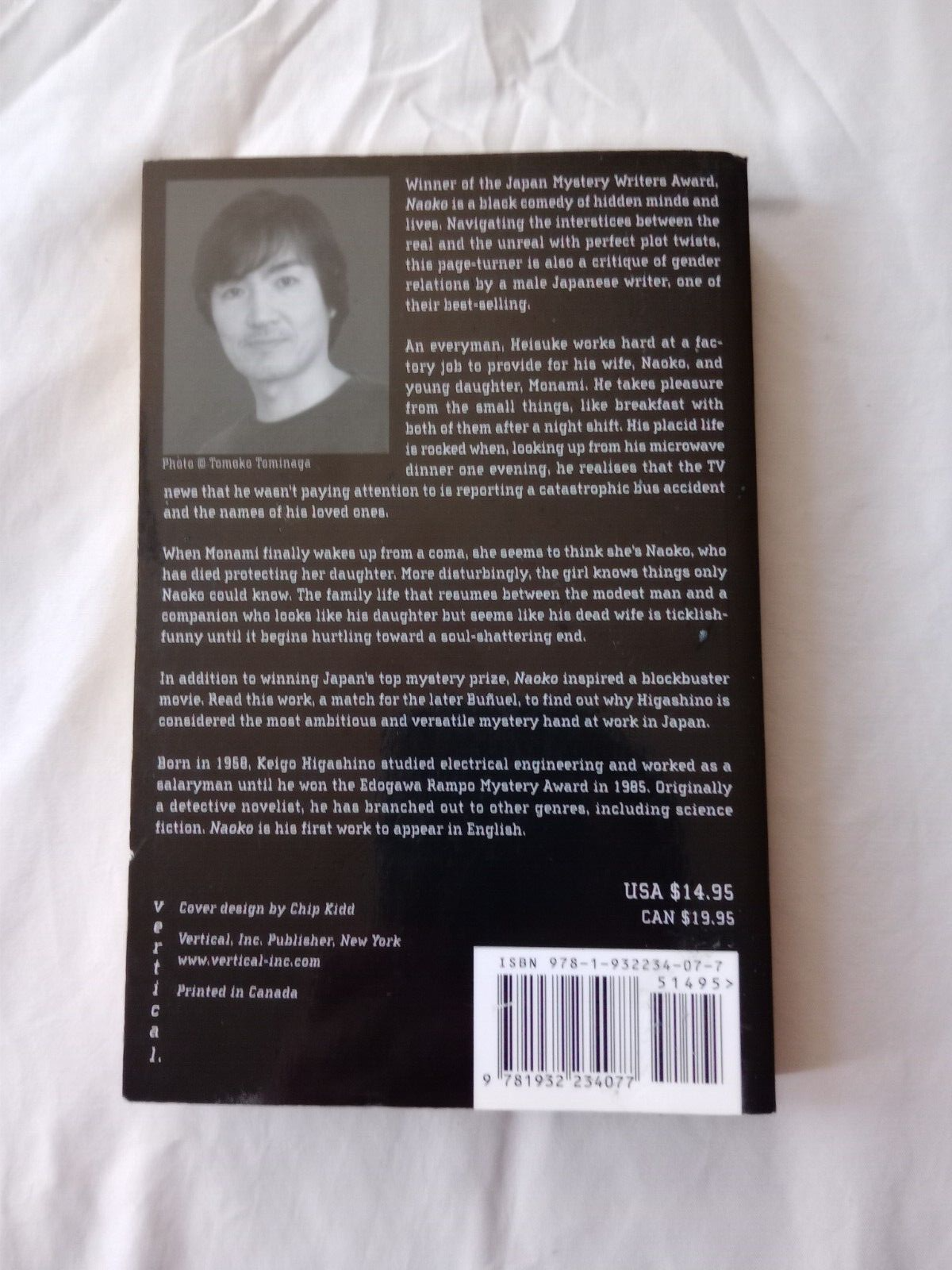The back cover of a black paperback book sits on a white, wrinkled cloth. The cover features a black-and-white photograph of the author, Keigo Higashino, in the top left corner, with photo credit to Tomoko Tomaga. The text announces that the book, "Naoko," has won the Japan Mystery Writers Award. The story is described as a black comedy exploring hidden minds and lives, navigating the boundary between the real and the unreal with perfect plot twists. It is also noted for its critique of gender relations by one of Japan's best-selling male authors.

The narrative centers on Kyousuke, a diligent factory worker who enjoys simple pleasures like breakfast with his wife, Naoko, and young daughter, Monami, after his night shifts. His ordinary life is shattered one evening when, while distractedly eating a microwave dinner, he notices a news report about a catastrophic bus accident that involves his loved ones. Naoko dies saving Monami, who, upon waking from a coma, disturbingly claims to be Naoko and knows things only Naoko would know. The book humorously yet poignantly explores the bizarre family dynamic that emerges as Kyousuke lives with a daughter who seems like his deceased wife, all leading towards a profound and unsettling conclusion.

"Naoko" has not only garnered Japan's top mystery prize but also inspired a blockbuster movie. This seminal work is a prime example of why Higashino, born in 1958 and originally an engineer who shifted to become an award-winning author, is celebrated as one of Japan's most ambitious and versatile mystery writers. Priced at $14.95 in the USA and $19.95 in Canada, the cover design is by Chip Kidd, and the book is published by Vertical Ink. The ISBN is 978-1-932234-07-7.